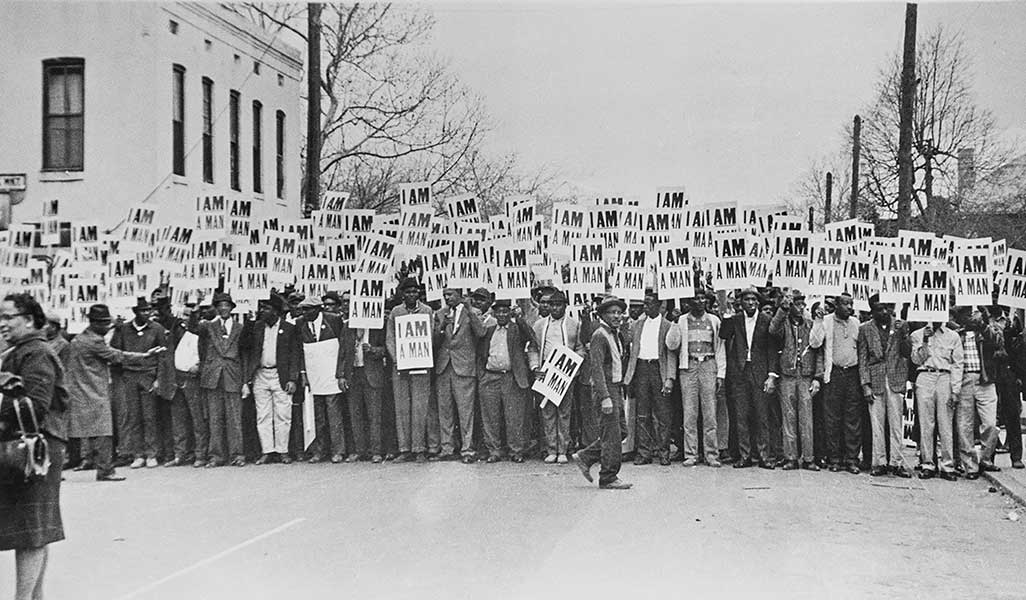This horizontally rectangular, black-and-white photograph, likely shot professionally using natural light, captures a poignant scene from a Civil Rights era protest. In the bottom left corner, a black woman facing away is discernible, wearing glasses, a skirt, a jacket, and carrying a purse. The main focus is a large group of African American men, clearly visible despite the limited palette of blacks, whites, and grays. They are lined up across a street, extending several rows back, each holding identical white protest signs that read "I AM A MAN." The backdrop features trees with sparse branches, a building in the top left corner, and telephone poles, reinforcing the setting as an American city during the 1950s or 1960s. The scene, steeped in historical significance, evokes a powerful message of dignity and recognition amidst the struggle for civil rights.